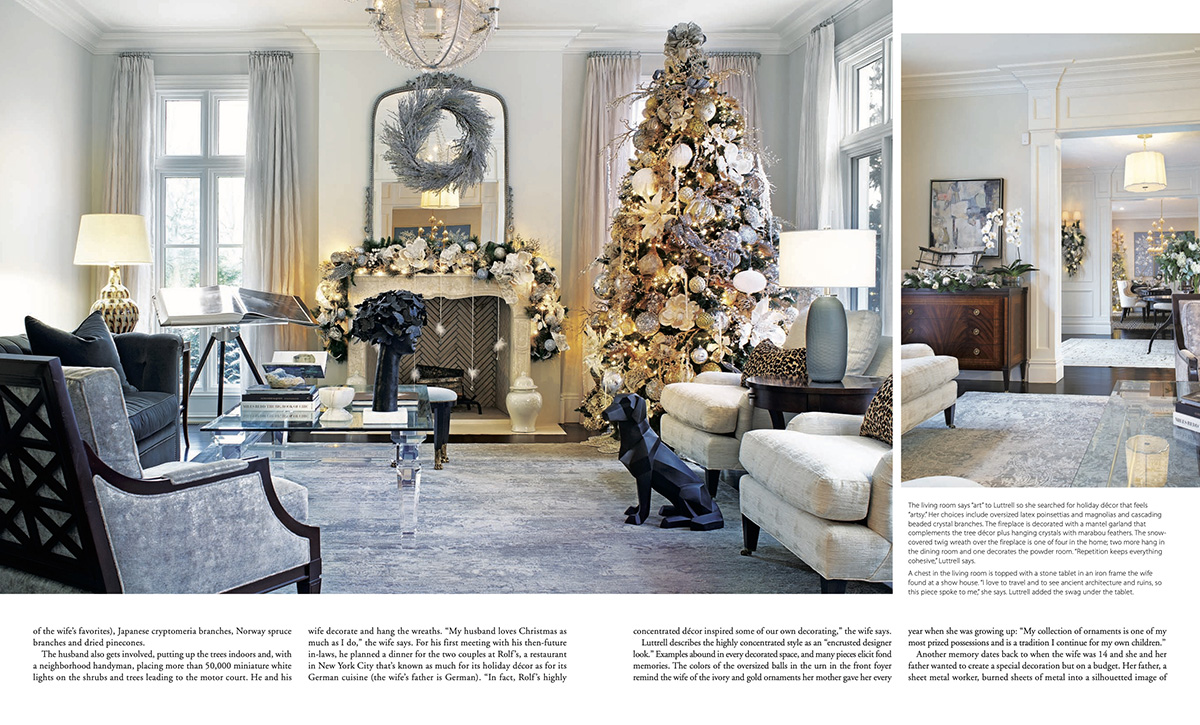The image is a magazine spread showcasing a detailed layout of a beautifully decorated living room during Christmas time. The left side of the spread, which takes up about two-thirds of the entire image, features a grand fireplace mantel adorned with a wreath and festive flowers. Above the mantel hangs a blue wreath, complementing the room's blue accents, which include a cozy blue chair and stylish blue lamps. Beside the mantel stands a tall Christmas tree decorated in blue, white, and gold ornaments, illuminated by bright yellow lights. The text highlights the wife's favorite ornaments: Japanese cryptomeria branches, Norway spruce branches, and dried pine cones. 

On the right side of the spread, taking up the remaining third of the image, is another view of the living room, possibly the same room, further showcasing the festive decor. The husband is noted for his involvement in the holiday preparations, decorating the trees indoors and, with help from a neighborhood handyman, placing over 50,000 miniature white lights on the shrubs and trees leading to the motor court. This shared passion for Christmas is a cherished aspect of the couple's lives, with inspiration drawn from grand holiday displays seen during a memorable dinner at Rolf’s, a New York City restaurant famed for its elaborate holiday decor.

The room itself is spacious and bright, featuring white walls, large windows, and a central glass table adorned with a black floral ornament. Beneath the images, text boxes provide further context and details, enhancing the overall descriptive narrative of this festive interior.